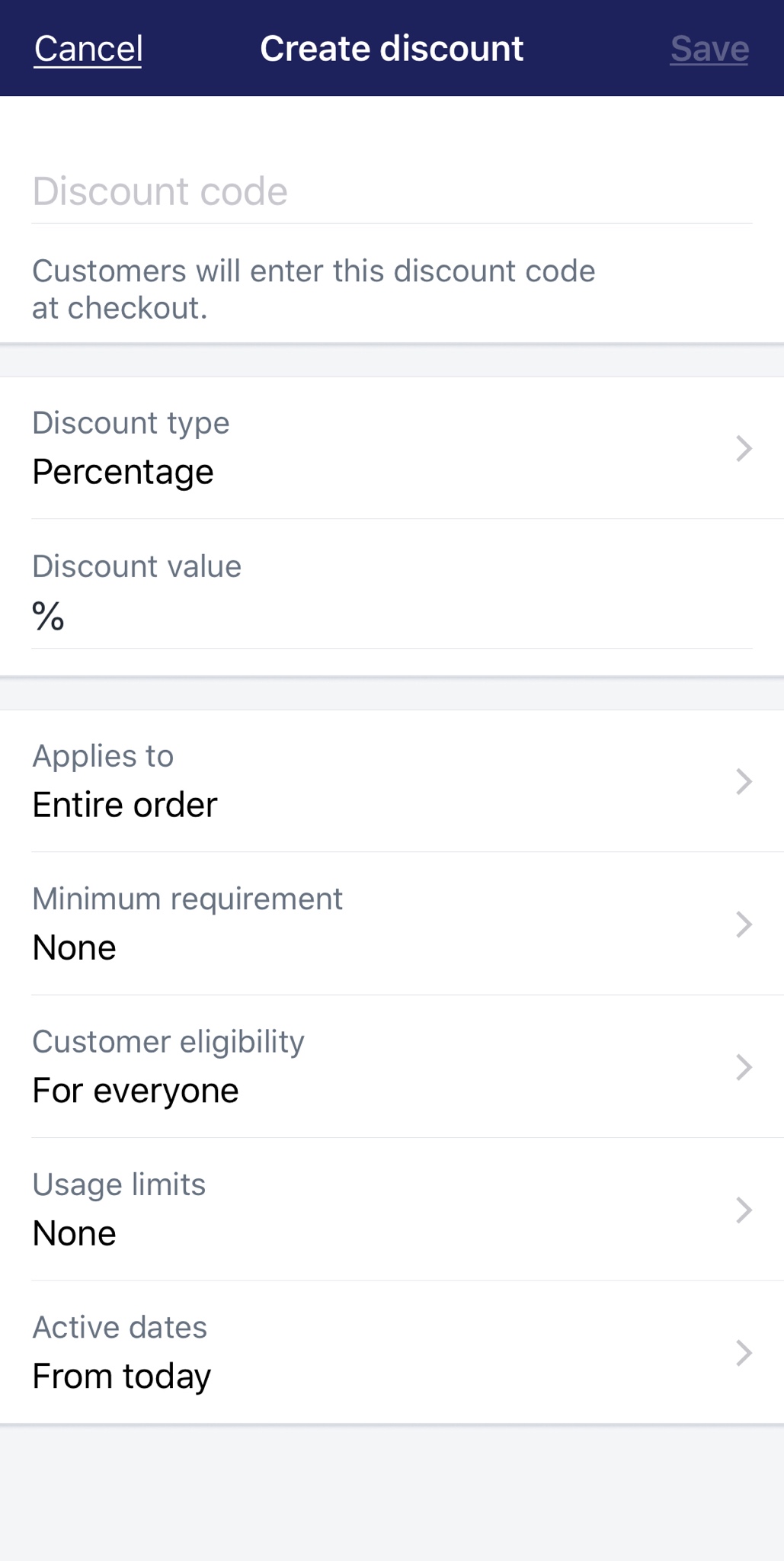The image depicts a mobile phone screen displaying a user interface for creating a discount. At the top of the screen, there is a dark blue header with a white "Cancel" option on the left, underlined. In the center, it reads "Create Discount," and on the right, the word "Save" is shown in gray with an underline.

Below the header on the left side, there is a section labeled "Discount Code" in gray, underlined. Directly below this, it says "Customers will enter this discount code at checkout," followed by a gray input box.

Further down on the left, there is a label "Discount Type" in gray text, followed by the option "Percentage" and a right-pointing gray arrow. Beneath this is another gray line separating sections.

Continuing below, the screen describes "Discount Value" in gray, accompanied by the word "Percentage" and another gray line below, leading to a gray input box for entering the discount value.

Next, the section "Applies To" indicates "Entire Order," with a gray arrow pointing to the right and a gray line beneath it. Below, "Minimum Requirement" is shown with the option "None," followed by another right-pointing gray arrow and gray line.

The following section, "Customer Eligibility," states "For Everyone" with a gray arrow pointing to the right, accompanied by a gray line below. Additionally, there is a "Usage Limits" section specifying "None," with the customary gray arrow and line underneath.

At the very bottom, the section "Active Dates" starts from "Today," with a gray line beneath it and a gray input box for selecting dates.

This comprehensive layout ensures that users can easily create and customize discount codes for their customers, with clear indications and organized fields.